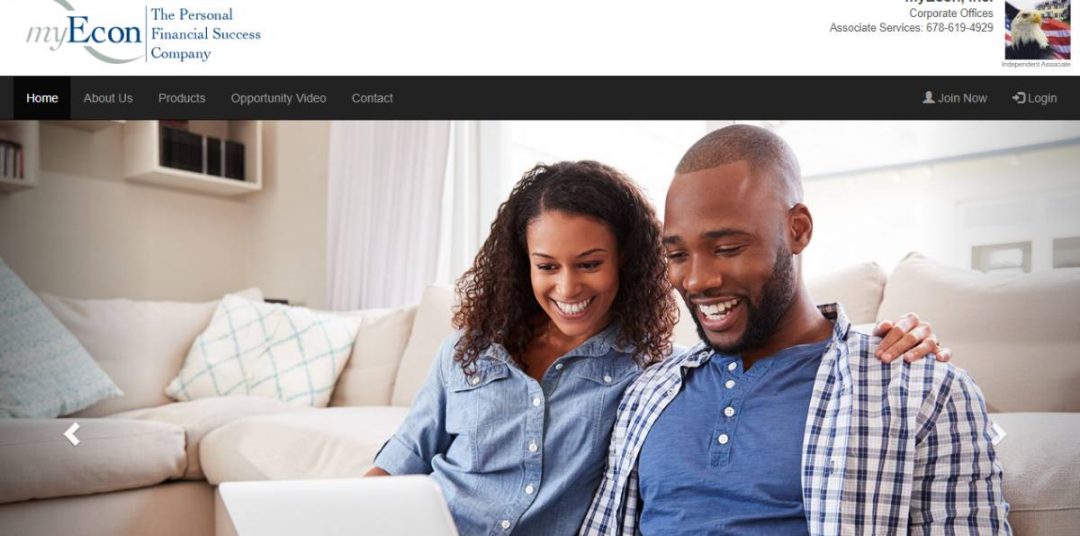The webpage of MyEcon, the personal financial success company, features a well-organized and visually appealing layout. In the upper left-hand corner, the company logo is displayed with the word "My" in light gray, lowercase, and italic font, followed by "Econ" in bright blue. A distinctive gray ribbon runs through the letter "E" in "Econ" and curves beneath the word, creating a dynamic visual effect. Adjacent to the logo, a vertical gray bar separates it from the slogan "the personal financial success company," written in bright blue text.

To the far right of the header, information is neatly presented with a contact phone number labeled "Associate Services" and a square photograph featuring an American eagle and an American flag. Beneath this header, a sleek black ribbon spans across the screen, housing navigational links: Home, About Us, Products, Opportunity Video, and Contact. On the far right of this ribbon, there is a people icon with the text "Join Now" next to it and a login option.

Dominating the main section of the webpage is a full-screen photograph of an affectionate couple seated on the floor of their living room. The man and woman, both with dark skin, are leaning against their sofa, intently focused on a silver laptop resting on the man's lap. The woman's arm is lovingly draped over the man's shoulder. Both are dressed in blue; the woman wears a blue denim blouse with a collar, while the man sports a blue Henley layered with a white and navy blue plaid shirt. The overall scene exudes a sense of comfort, connection, and shared financial empowerment.